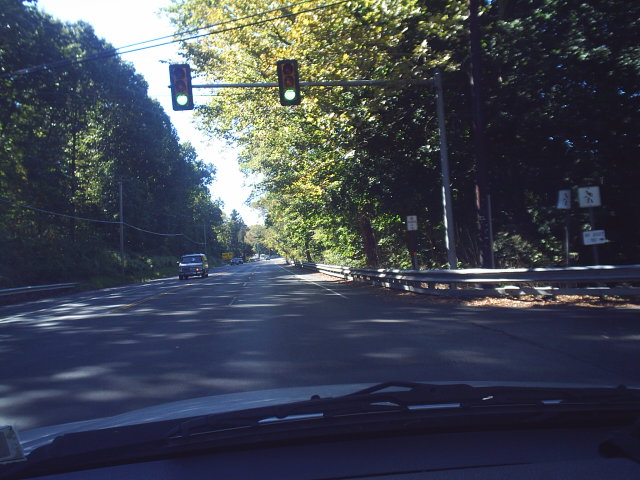The image depicts a daytime view from inside a car, looking out through the front windshield. At the bottom of the image, parts of the car’s black dashboard, gray or silver hood, and windshield wipers are visible. Ahead, the black asphalt road with three lanes—two heading in the driver's direction and one for oncoming traffic—stretches forward. In the distance, a green traffic light mounted on a gray pole shows green in both directions. On the left, an oncoming van approaches, with smaller cars following in the background. Both sides of the road are lined with tall, leafy trees, some with green and others with yellowing leaves, hinting at a rural or forested area. A gray metal barrier runs along the road's edge, and various white signs with black images and words, though unclear in detail, can be seen, including some that resemble pedestrian prohibition signs. Crisscrossing power lines hang overhead, and the sky above appears a whitish blue.